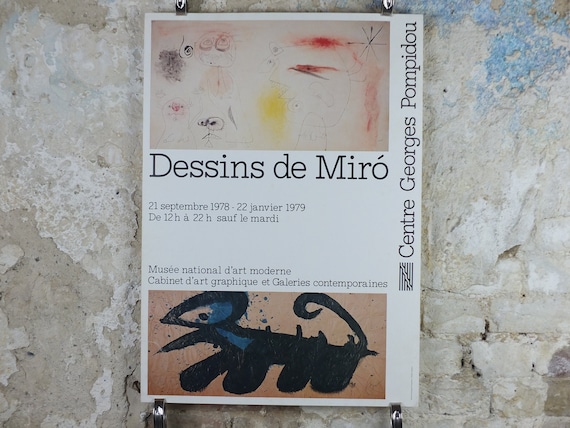The image depicts a pass or ticket for an art exhibit, placed on a countertop with a granite-like appearance showcasing shades of gray, white, and blue. The pass, secured by metal hooks and set on a cream-colored background, features two distinct abstract art pieces. The top artwork displays a chaotic mix of colors with random sprays of red, yellow, and black, accompanied by faint lines and possible stick figure imagery. The bottom piece resembles a childlike drawing of a creature with four legs, a curved tail, and an oval head with blue and black details. Prominently, the text "Dessins de Miró" is displayed in large black letters, with a smaller inscription below noting "Musée National d'Art Moderne."